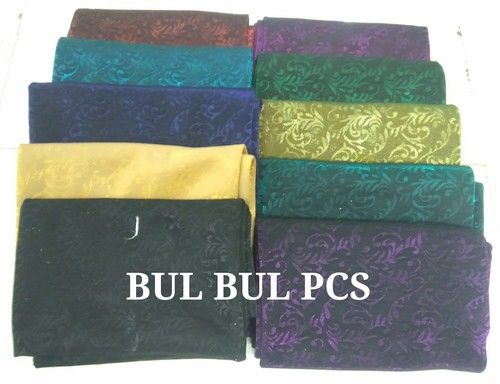The image showcases an array of 10 pieces of textured fabric arranged in two columns, extending from the front to the back. Each piece of fabric is folded in a rectangular shape and is several layers thick, featuring a delicate curlicue pattern with a subtle reflective quality. The left column displays fabrics in the following sequence from front to back: navy blue, ivory, midnight blue, deep turquoise, and burgundy. In the right column, the fabric colors are lavender, turquoise, green, deep green, and purple. Across the front of this vibrant display, prominent white text spells out "BULBULPCS." The background is completely white, emphasizing the colorful and intricately designed fabrics that evoke a sense of an advertisement or promotional display.